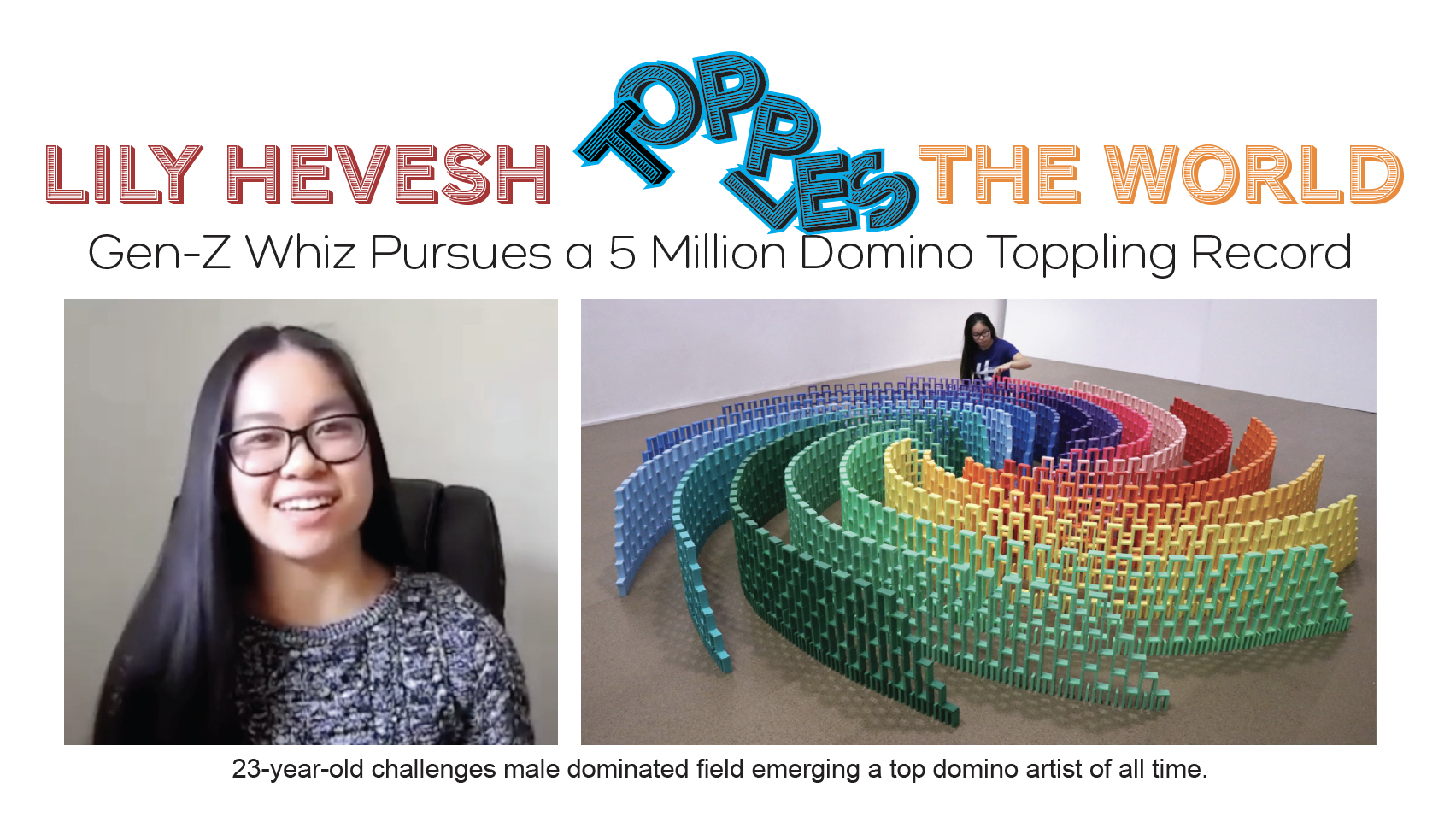The image is a composite of two separate visuals placed side by side with a noticeable gap in between. The left portion features a young woman seated in a black chair. Her outfit, though partially obscured, appears to be a top with a mix of blue, black, and white colors. Her hair falls gracefully over her left shoulder, and she is wearing black glasses. A warm, friendly smile adorns her face.

To the right of her, there is a vivid display of various twigs or branches that resemble colorful fences. The colors range across a vibrant spectrum, including neon pink, red, orange, bright golden yellow, light green, green, periwinkle, light blue, and several shades of purple up to violet.

Above this vibrant array, text is displayed in a sequence: "Red Lily Hevesh" at the top, followed by "Topples" in the middle, and finally, "The World" at the bottom. This typography adds context and a sense of dynamic action to the image.